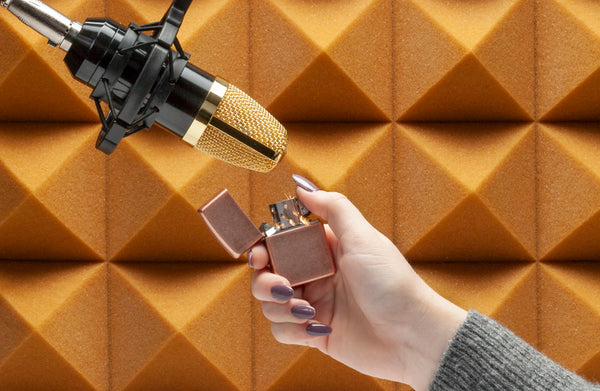This detailed color photograph captures a close-up scene possibly set in a recording studio. The main focus is on a woman's pale, manicured hand emerging from the lower right-hand corner, adorned with purplish-gray mauve painted nails and wearing a gray sweater that extends to her wrist. She's holding a rose gold or copper-colored Zippo lighter, which is sparking but not yet lit, revealing its silver inner mechanism. 

The lighter is positioned in front of a microphone that descends from the upper left-hand corner on a silver boom arm. The microphone’s body is black with a chrome stand, and it has a distinctive gold mesh grill with a black stripe. The background is lined with orange, pyramid-shaped acoustic foam, reinforcing the studio setting with its sound-insulating properties. The intricate details of the hand, lighter, and microphone are prominently featured, emphasizing the intent and careful composition of the scene.